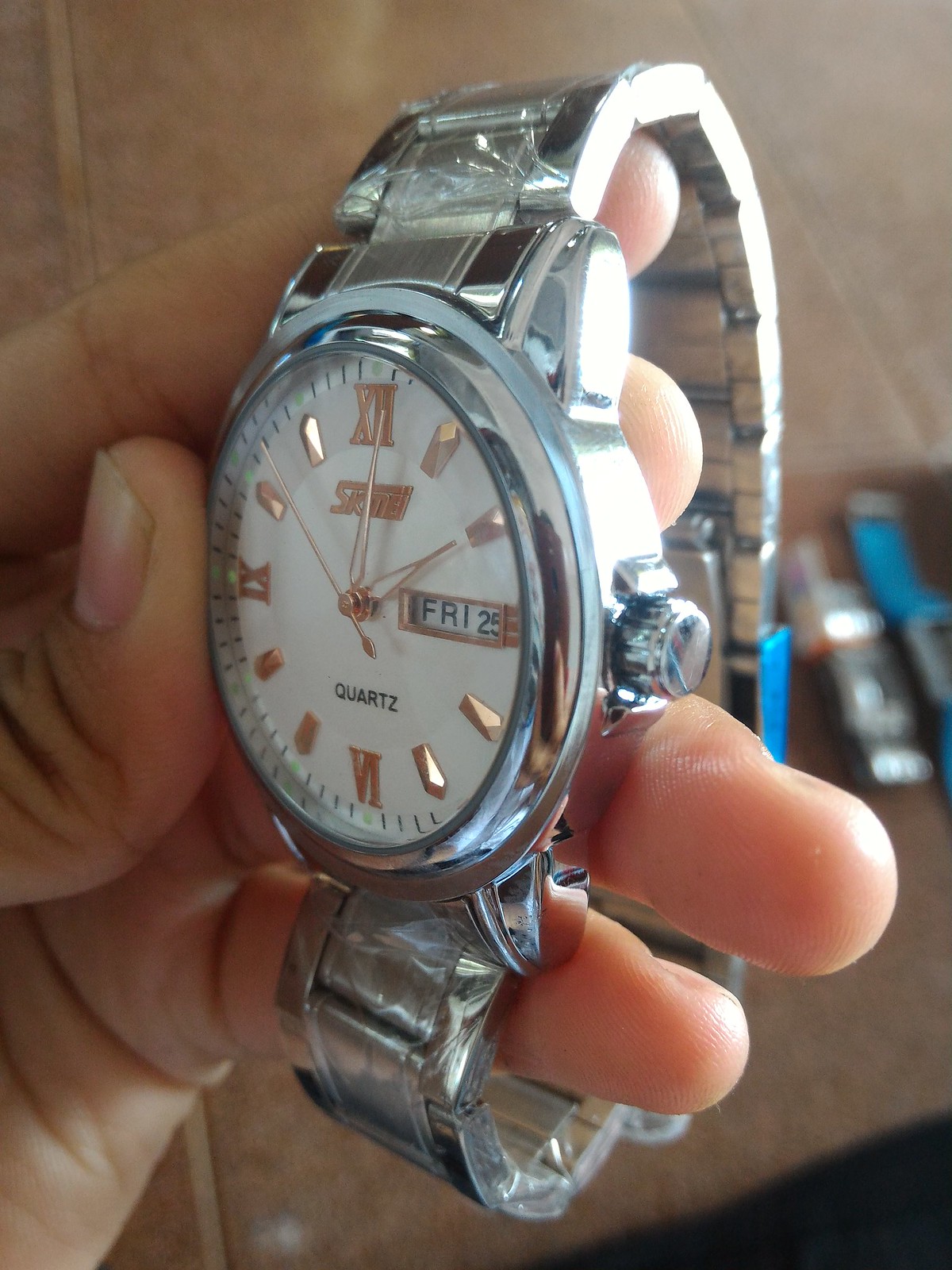A close-up image captures a left hand delicately holding a wristwatch by its silver metal band. The watch features a polished silver case, and its winding crown is prominently visible on its right side. The white dial of the watch is adorned with elegant gold Roman numerals and matching gold hands. At the 3 o'clock position, there is a rectangular window outlined in gold, displaying the day "Friday" and the date "25". The word "Quartz" is printed in black letters on the watch face. Although the brand name is present below the 12 o'clock marker, it remains unreadable due to the angle at which the watch is held. The background consists of a brown table, with some indistinct white, blue, and black objects positioned off to the right.